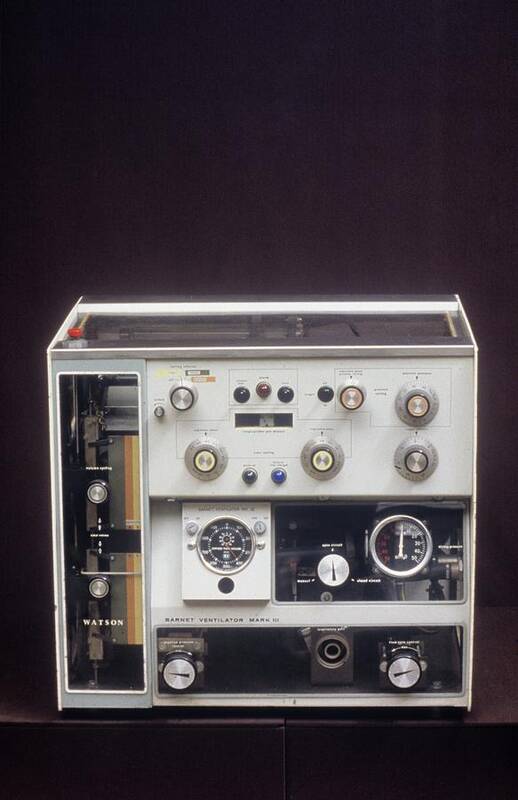This photograph depicts an older piece of industrial technology, identified as a "Barnet Ventilator Mark III," possibly dating back to the 1960s or 70s. The apparatus has a boxy, almost cube-like shape and is predominantly white with silver knobs. The device showcases various analog dials and gauges prominently in the middle, with numbers indicating different parameters. 

The front panel features multiple indicator lights—green, red, and blue—and there are multiple knobs for adjustments. To the left side of the device, a clear panel with two additional knobs is visible, with the name "Watson" inscribed in white below them. The bottom front of the unit includes a couple of knobs and what appears to be a port or plug. 

Overall, the device is placed against a brown background, possibly a table, although the exact surface is obscured within the photograph, which has a slightly blurred, low-resolution quality.